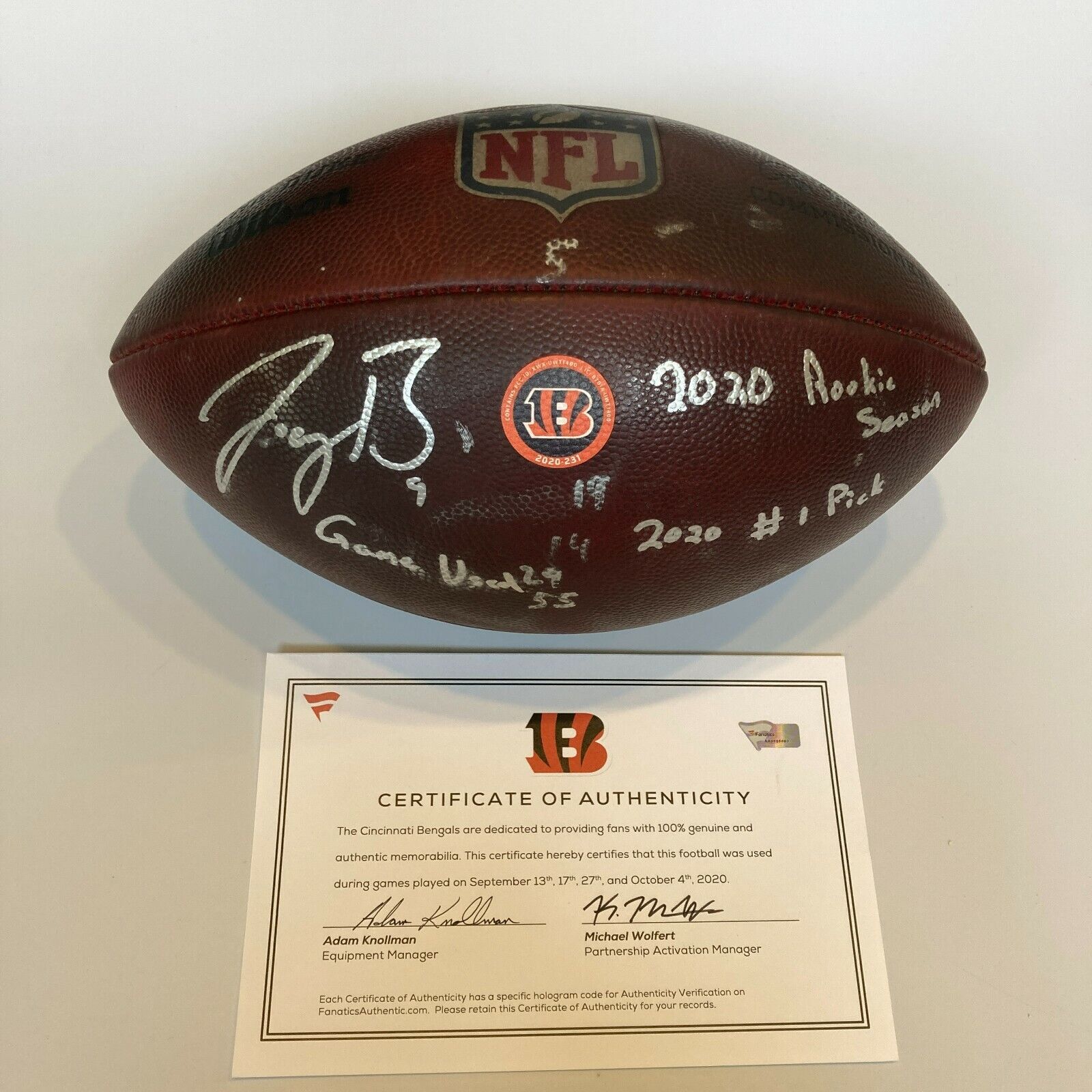The image is a vertically rectangular, staged, full-color photograph taken indoors under artificial lighting, featuring an old, dark brown leather football against a gray background that transitions from darker at the top to lighter at the bottom. The football is emblazoned with the NFL logo, a red, white, and blue shield near the top, and the word "Wilson." Several signatures, the number “5” in white, and the year "2020 rookie season" are prominently marked on its surface. Below the NFL logo, an orange circle logo with a black and orange striped "B" identifies the Cincinnati Bengals. Beneath the football sits a certificate of authenticity, which certifies the ball was used during games on September 13th, 17th, 27th, and October 4th, 2020, and includes signatures from Adam Nolman, Equipment Manager, and Michael Wolfert, Partnership Activities and Activation Manager. This football is authenticated as game-used from the 2020 rookie season and indicates it belonged to the number one draft pick, adding significant detail about its provenance and importance.